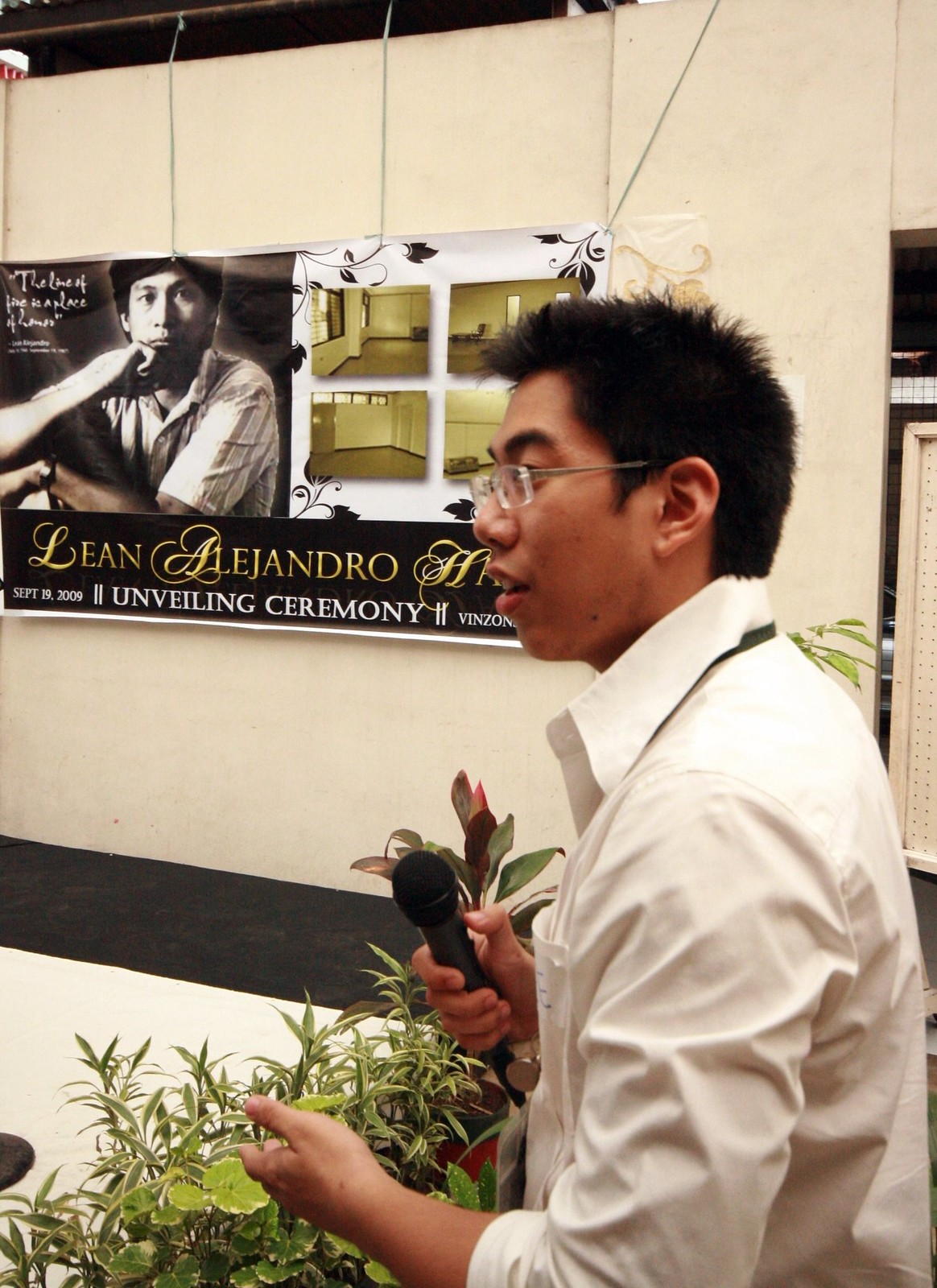In this photograph, captured indoors, we see an Asian man positioned at the bottom right of the image, holding a microphone while speaking at a ceremony. The man, who appears from the waist up, has spiky, short, dark hair and wears glasses along with a long-sleeve, white-collared shirt. His left arm is bent at the elbow and his hand gestures outward as he looks towards the left side of the image. His right hand, partially obscured by his body, holds the microphone. 

In the foreground, a tiled floor is visible and just above it, there are small potted plants with their green leaves rising up. In the background, a light tan wall displays a banner with the heading "Lean Alejandro Unveiling Ceremony" in yellow text on a black strip at the bottom. The banner prominently features a picture of an Asian man, likely Lean Alejandro, on the left side, and four smaller pictures of an empty room on the right side. Additional text and details are partially obscured by the man’s face, but one can make out the date September 19, 2009. The entire scene is illuminated indicating it could be either daytime or nighttime, creating an atmosphere set for a ceremonial event.